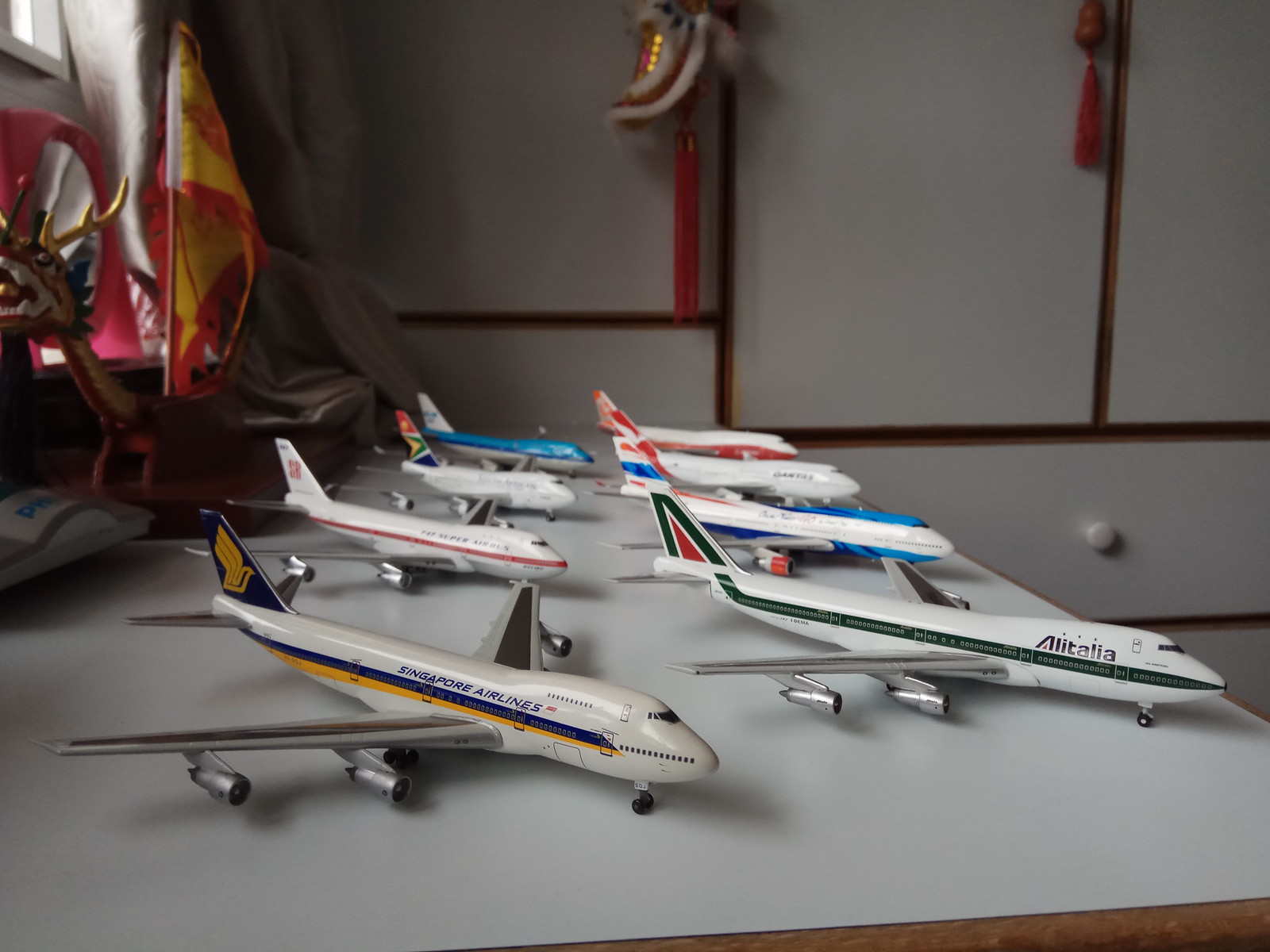The photograph showcases a detailed collection of eight model Boeing 747 airplanes, meticulously arranged on a white table with a wood-banded trim. These models, distinguished by different liveries representing various airlines, including Singapore Airlines in silver, blue, and yellow, and Alitalia in green and white, are all oriented diagonally toward the bottom right corner of the image. The room, possibly a bedroom or garage, features white cabinets and drawers with dark brown accents in the background, accented by distinctive white knobs. Soft light filters in from a window in the upper left corner, casting a gentle glow over the scene. Additional notable items include a small yellow and red desk-sized flag, likely representing Spain, and a decorative red and gold dragon figurine to the left of the desk. The composition creates a sense of organized display, capturing both the ambiance of the room and the precision of the model collection.